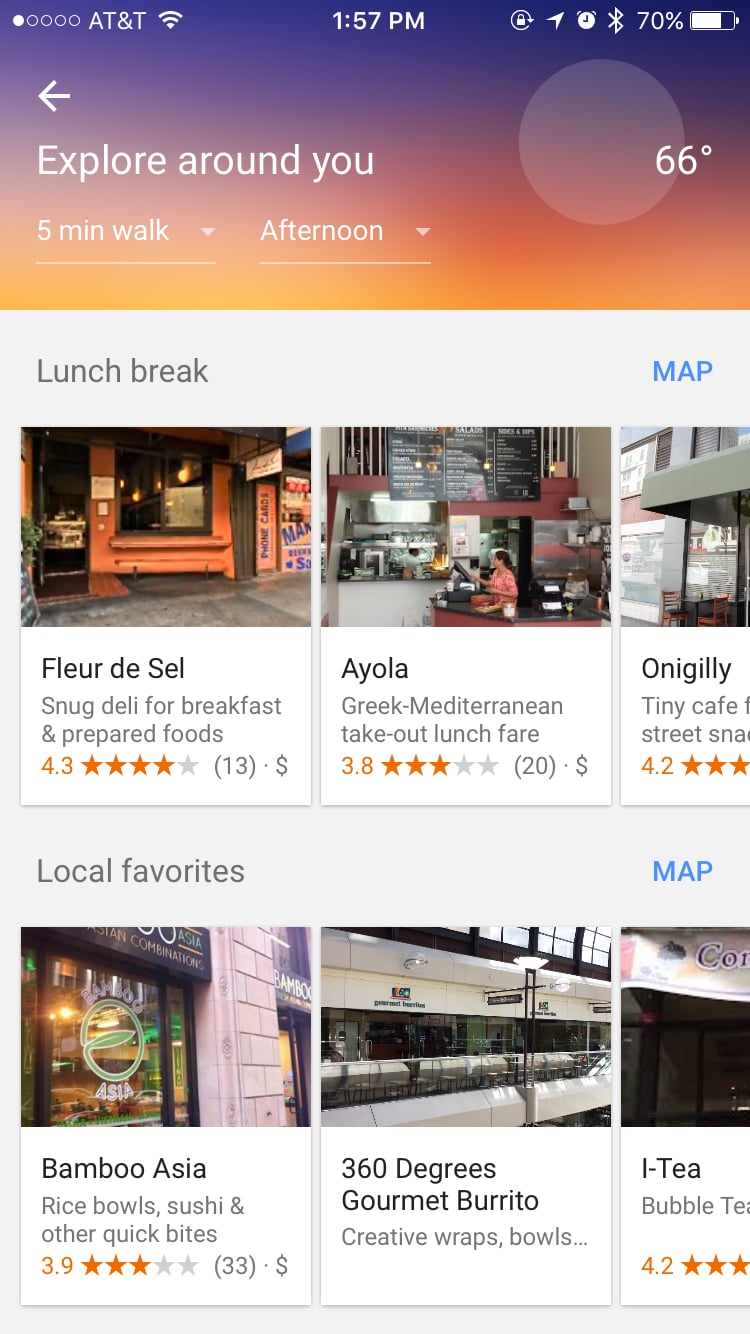This is a detailed screenshot from a cell phone. At the top, a gradient rectangle spans horizontally, starting with a deep purple at the top corner, fading into lighter purple, transitioning into a rosy orange, and finally blending into a light tangerine orange. The text within this gradient bar is white. 

In the upper left corner, there are five circles: the first one is white, while the remaining four are purple outlined in white. Adjacent to these circles is the text "AT&T," followed by a Wi-Fi signal icon. Centered at the top, the time "1:57 p.m." is displayed. On the far right, various icons indicate the signal strength, Bluetooth connectivity, and battery level.

Below this gradient header, there is a directional arrow pointing to the left. Further down, the text "Explore around you" is prominently displayed, followed by a marker that indicates a "Five-minute walk." To the right of this marker is the word "Afternoon" and a faint circle displaying the temperature, "66 degrees."

Directly underneath on a white background, there are two sections: "Lunch Break" on the left and "Map" on the right. Below this, three images of different dining spots are presented in sequence. The first image showcases a storefront for "Fleur de Sel," described as a snug deli for breakfast and prepared foods, rated 4.3 stars based on 13 reviews. The second image shows the interior of "Iola," a Greek and Mediterranean takeout spot with a 3.8-star rating. The third image features the exterior corner of another establishment.

Continuing downward, the text "Local Favorites" appears on the left, with "Map" on the right. Immediately below this, there's an image of an Asian restaurant's storefront labeled "Bamboo Asia," offering rice bowls, sushi, and other quick bites, rated 3.9 stars from 33 reviews. This is followed by an image of "360 Degrees Gourmet Burrito," accompanied by the text "Creative wraps and bowls."

This detailed description encapsulates the contents and layout of the screenshot, providing a vivid depiction of the cell phone display.